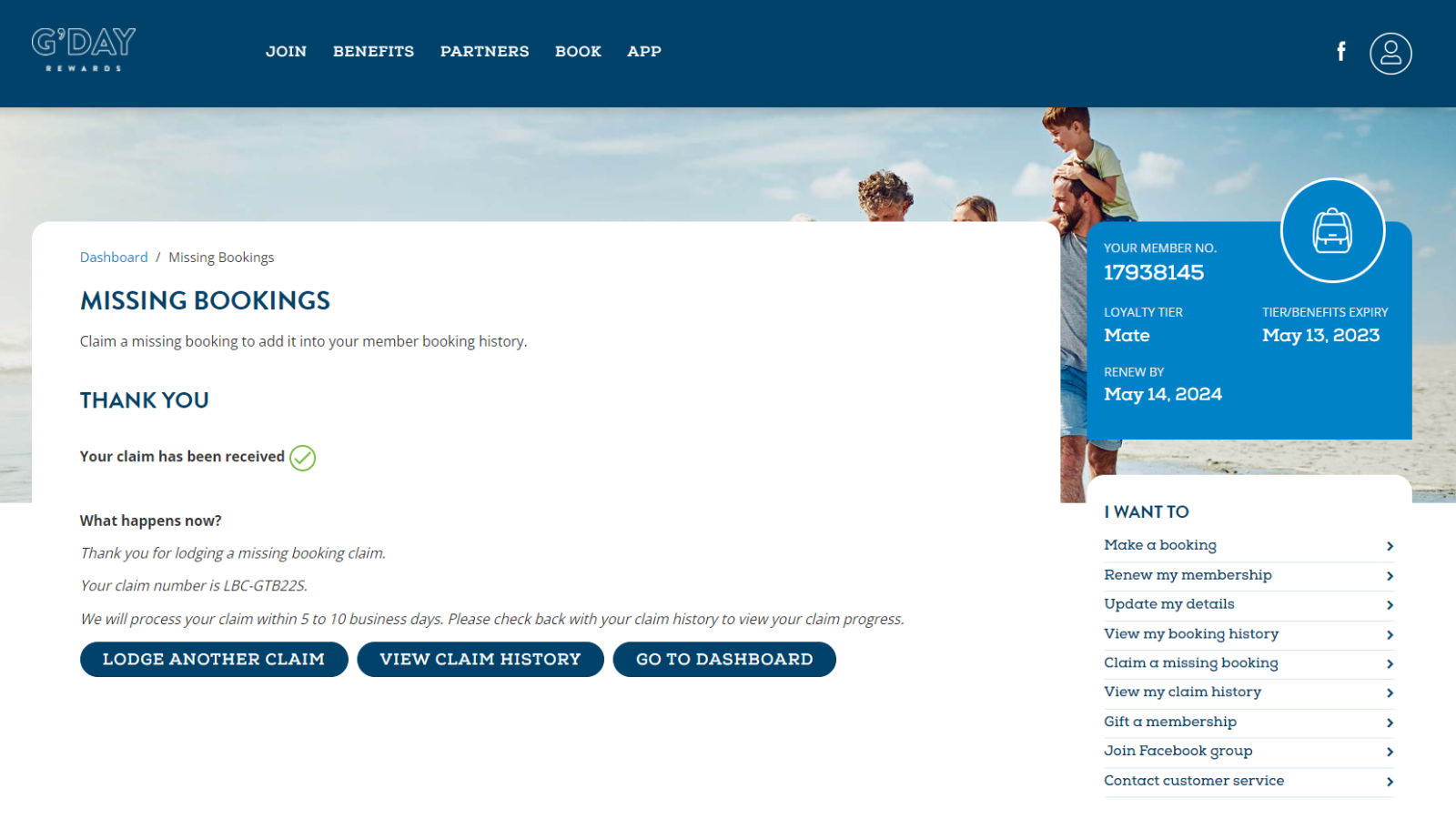**Image Description: Digital Dashboard Overview for a Reward Program**

The image features a sleek digital dashboard on a navy blue background. At the top left corner, the text "G'day" is prominently displayed in all caps, followed by the word "Rewards," both in white font. To the right, five tabs are visible, labeled "Join," "Benefits," "Partners," "Book," and "App." On the extreme right, there is a shortcut for the Facebook logo next to a user profile picture.

Below this, there is a cut-out image of a cheerful family. The father is giving his young son, who appears to be around five or six years old and wearing a light green shirt, a piggyback ride. The family, likely Caucasian, is set against a sunny backdrop with faint clouds on the horizon.

To the right of the family photo, text on a light blue background reads "Your Member Number" alongside a logo of a backpack enclosed in a circle. The member number is 17938145. The loyalty tier is labeled "Mate," with renewal due by May 14, 2024, and tier/benefits expiry on May 13, 2023.

To the left of the loyalty information is a predominantly white section with the text "Dashboard / Missing Bookings." Below this header, a highlighted section reads "Missing Bookings," with instructions to "Claim a Missing Booking to add it into your member booking history."

Further down, a bold "Thank You" is followed by the message "Your Claim has been received," accompanied by a green checkmark. A question below—"What Happens Now?"—is answered with: "Thank you for lodging a Missing Booking Claim, your claim number is LBC-GTB22S. We will process your claim within five to ten business days; please check back with your claim history to view your claim progress."

At the bottom, three blue pill-shaped buttons offer actions: "Lodge Another Claim," "View Claim History," and "Go to Dashboard."